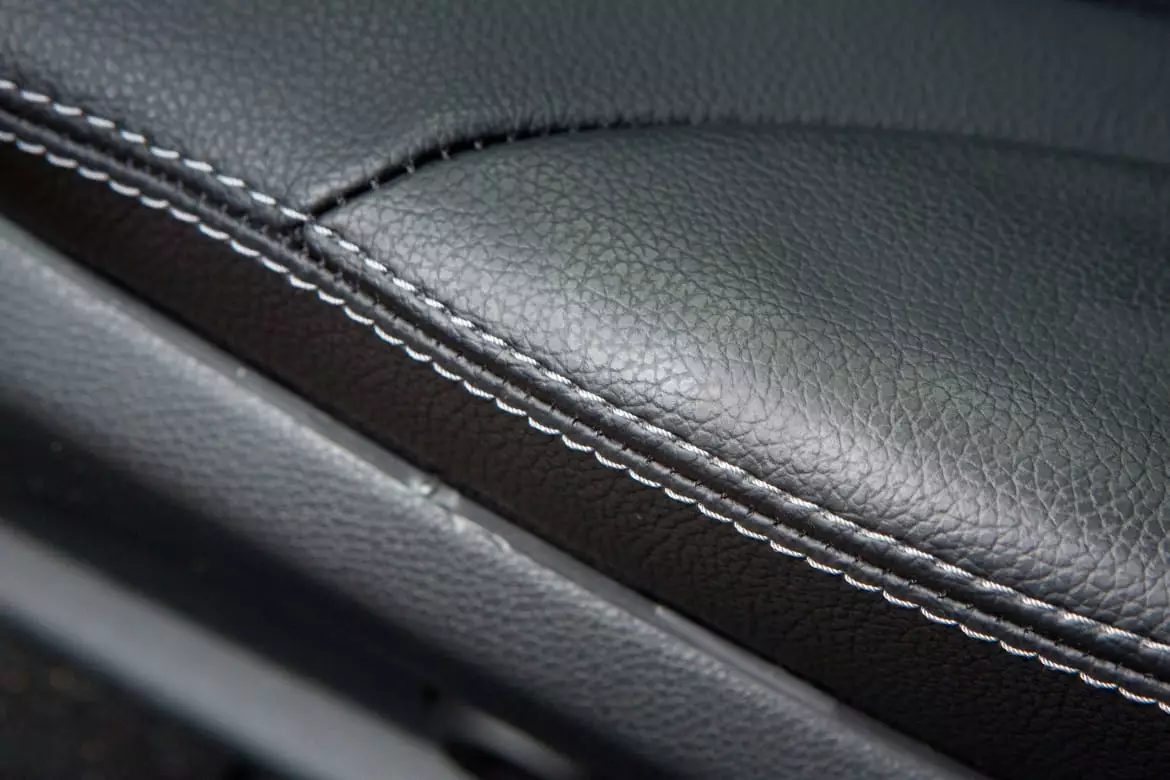This image is a very close-up, horizontal, rectangular photograph of what seems to be an upholstered black leather item, possibly a woman's purse, luggage, or a car seat. The leather, which has a textured surface, features a prominent seam with detailed white stitching. The seam, comprising two rows of white threading, runs diagonally from the upper left to the bottom right. Just above the halfway mark of the image, a horizontal crease in the leather is visible. Additionally, two gray plastic-like bars, approximately an inch thick and with a rough surface, traverse from the upper left to the lower right. These bars might serve as connectors, reinforcing the structural integrity of the item by linking the pieces together.